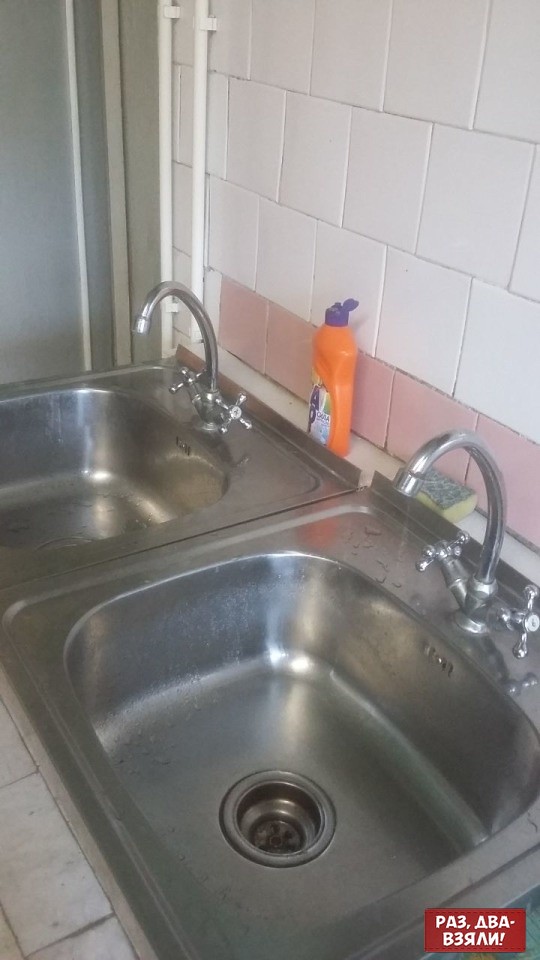The photograph showcases a kitchen sink area featuring two large, industrial-looking stainless steel sinks positioned side by side in a tiled countertop. Each sink has its own faucet with dual temperature controls. Centrally located between the sinks is an orange detergent bottle with a purple lid, and nearby is a well-used yellow scrubber with a green pad. The backsplash is composed of white tiles at the top and a distinctive pink tile border at the bottom, altogether suggesting the need for re-grouting. In the lower right corner of the image, there's a red square watermark with backward lettering "PA3-ABA-B," possibly in a non-English language. The setting hints that the sink might be adjacent to a window.